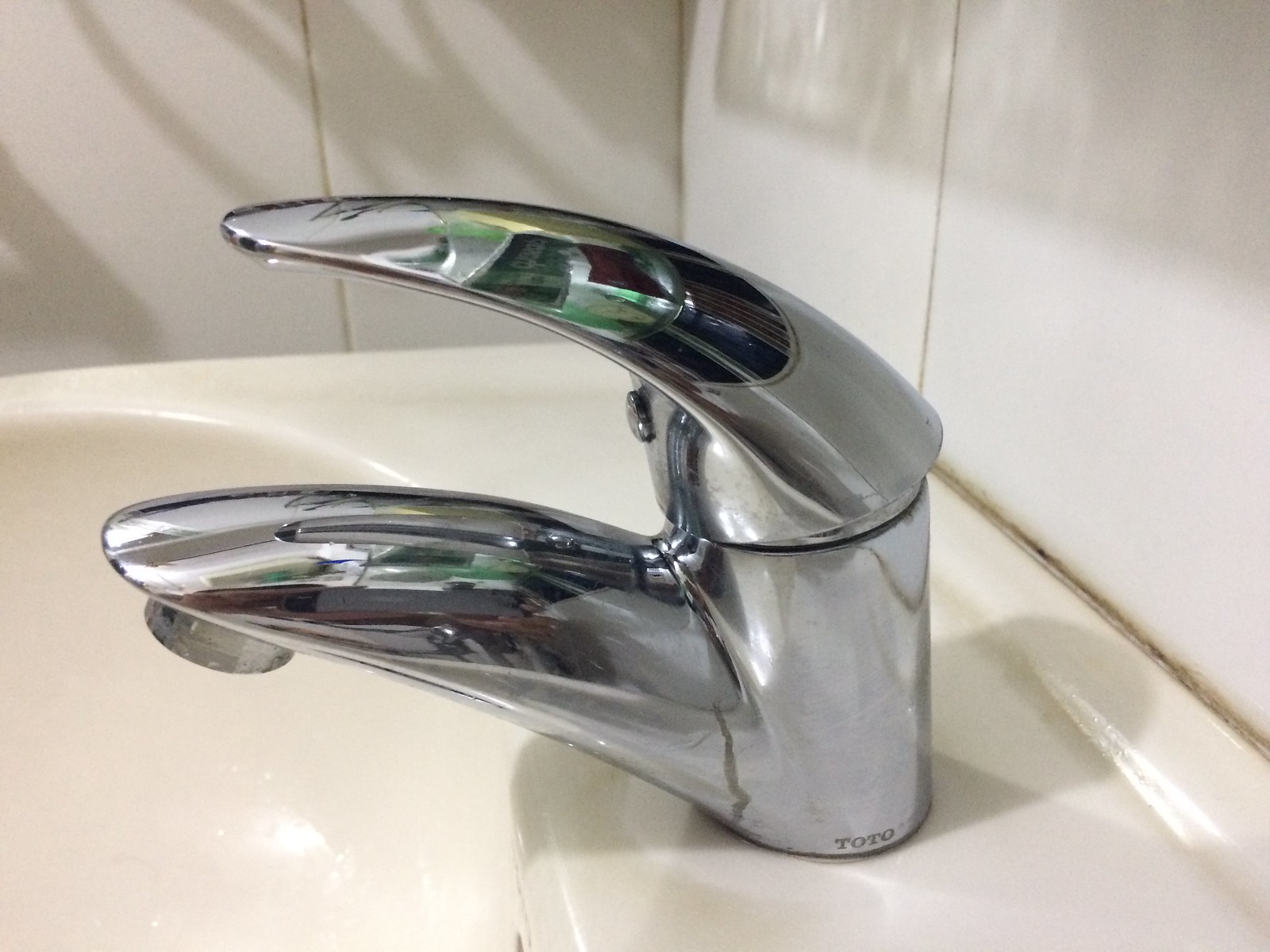A close-up image of a sleek, modern metal faucet by Toto, featuring a single lever handle positioned above a pristine white sink. The faucet's spout elegantly arches forward, allowing for easy water flow control. The background showcases a clean, white wall that complements the minimalist aesthetic of the scene. The design suggests the lever can be turned left and right to adjust the water temperature, embodying both functionality and style.